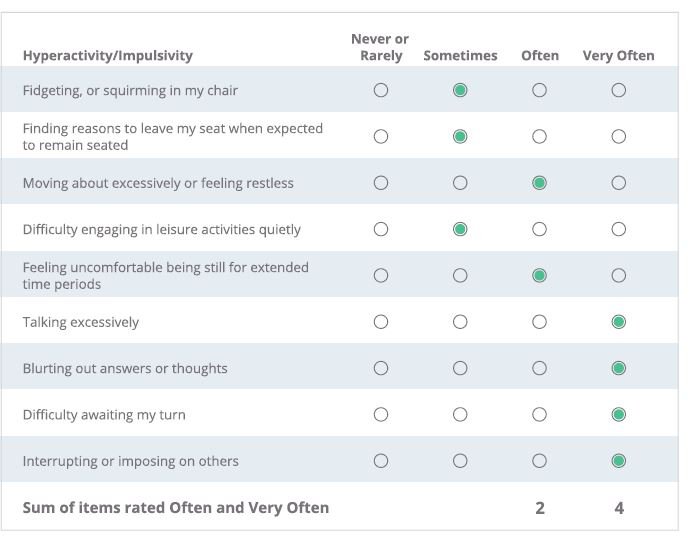The image depicts a detailed assessment form for hyperactivity-impulsivity, organized in a grid layout for evaluating various behaviors. 

**Caption:**

At the top left corner, the header reads "Hyperactivity-Impulsivity," followed by columns labeled "Never or Rarely," "Sometimes," "Often," and "Very Often." Each row under this header lists a specific behavior and its corresponding frequency, indicated by a green filled box. 

Starting from the top row, the behavior "Fidgeting or squirming in my chair" is marked under "Sometimes" with a green box. Similarly, "Finding reasons to leave my seat when expected to remain seated" is also marked "Sometimes" in green. 

Next, "Moving about excessively or feeling restless" is indicated as "Often" with a green box. The behavior "Difficulty engaging in leisure activities quietly" is marked "Sometimes" in green. "Feeling uncomfortable being still for extended periods" is marked "Often" with a green box.

For the rows listed under "Very Often," "Moving excessively" is marked with a green box. Additionally, "Blurting out answers or thoughts," "Difficulty awaiting my turn," and "Interrupting or imposing on others" all have green boxes under "Very Often." The final behavior, "Interrupting or imposing on others," is also checked as "Very Often" in a green circle.

At the bottom of the form, in black text, it states: "Sum of items rated Often and Very Often," followed by a tally showing '2' behaviors under the "Often" column and '4' behaviors under the "Very Often" column.